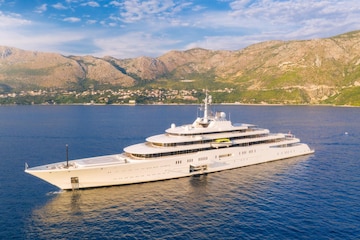This photo, taken from a slightly elevated angle, captures a large, white superyacht gliding across a vividly blue body of water. The yacht, which appears enormous, features three levels with numerous windows, and although it's not bustling with activity, its sleek design stands out in the serene setting. The background reveals a scenic coastline, adorned with a mix of small houses and buildings that suggest a small town. Beyond the town, rolling hills and rugged mountains punctuate the landscape, covered sporadically with patches of green grass but sparse on trees. Above, the sky is a clear, majestic blue, dotted with fluffy white clouds, amplifying the brightness of the scene. The yacht's reflection shimmers on the sunlit water, completing this picturesque moment of tranquility.